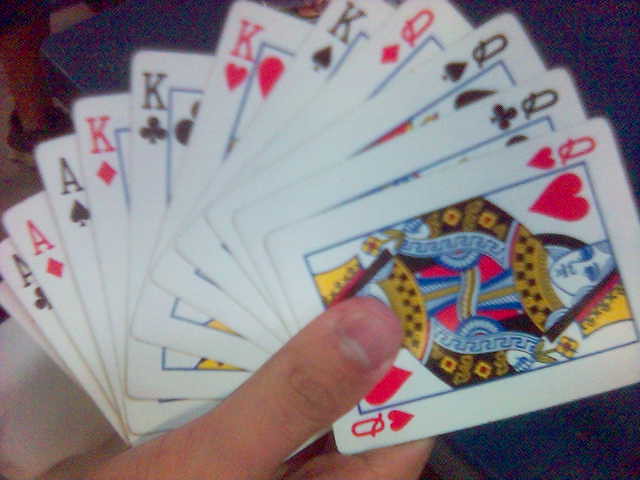A close-up photograph capturing a person's thumb and index finger holding a fan of playing cards. The visible cards are arranged in a neat sequence, featuring four Queens (Queen of Hearts, Queen of Clubs, Queen of Spades, Queen of Diamonds), four Kings (King of Spades, King of Hearts, King of Clubs, King of Diamonds), and three Aces (Ace of Spades, Ace of Diamonds, Ace of Clubs). There is also a twelfth card, partially cut off from the frame, leaving its identity a mystery. The cards are prominently displayed toward the camera, suggesting a photo opportunity rather than an actual game in progress. The meticulous arrangement and presentation of the cards create a visually appealing and intriguing image.